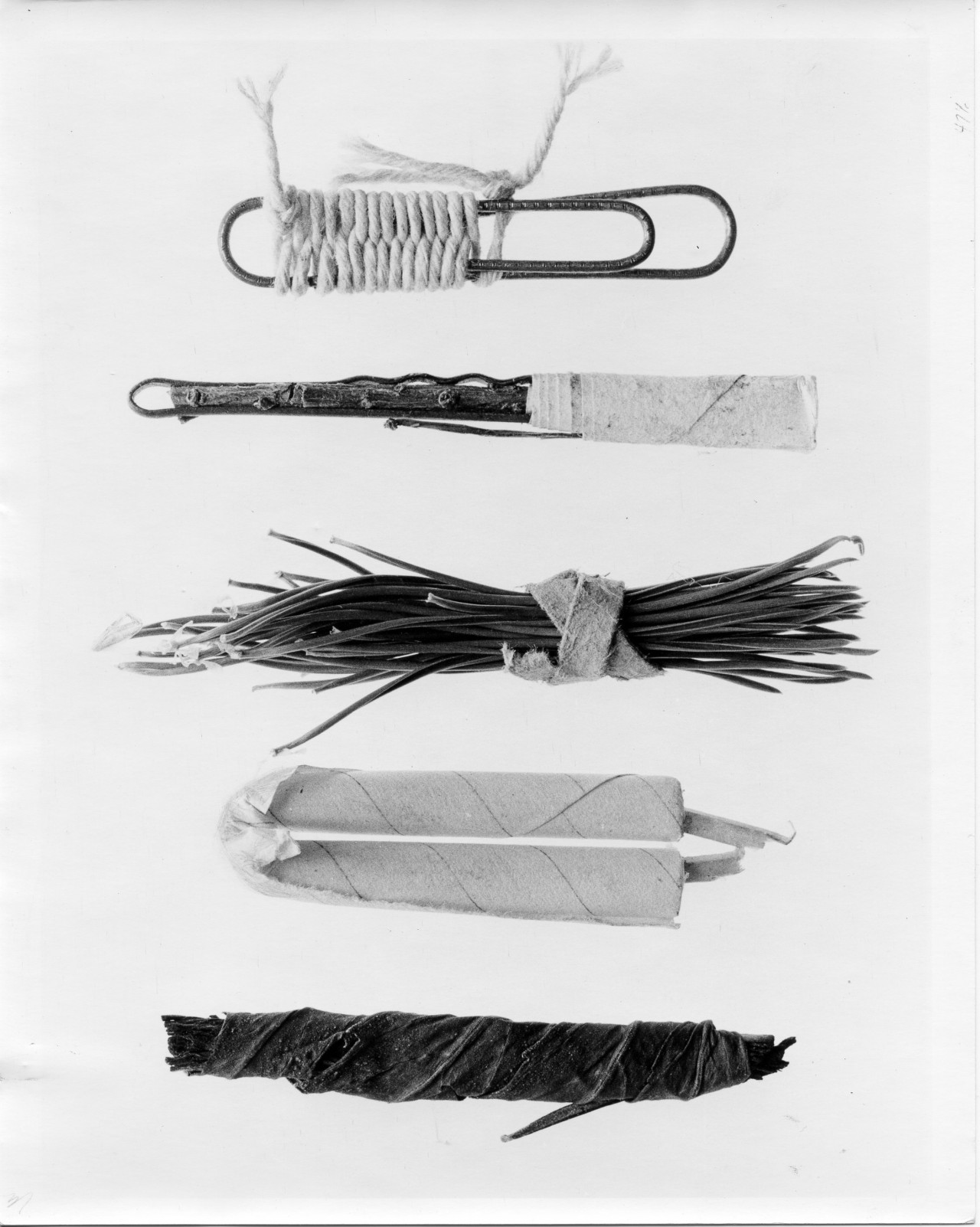This black and white photograph features five peculiar items arranged vertically, each uniquely bundled and bound. At the top, a paperclip is intricately woven with string, creating a detailed pattern reminiscent of ceremonial or battle adornments. Below it, a wooden-handled object is attached to a white cylindrical tube, possibly made of cardboard. The third item appears to be a knot of stems or chives, bound together by a thick tape that has a rope-like texture. Following that is a bent cardboard tube, akin to a paper towel roller, with something tied around its middle. Finally, at the bottom of the image, a bundle of sticks is wrapped in black cloth, adding to the eclectic mix of the five objects against a white backdrop.